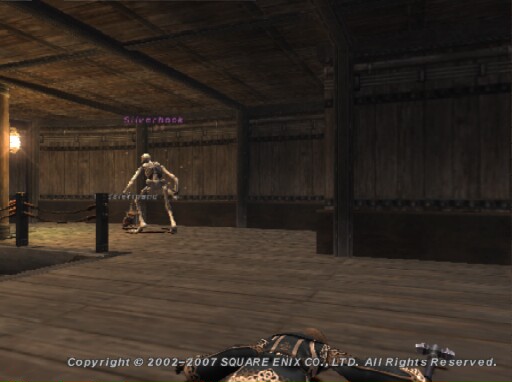A detailed image from a Square Enix game, showcasing an environment steeped in rich textures and intricate details. The foreground features a striking wood floor composed of a variety of wooden boards, each contributing to a mosaic of natural hues and grains. In the background, vertical wooden panels rise up, flanked by imposing dark pillars that add depth and a sense of grandeur to the scene. Notably, the rear bar is inscribed with "Copyright 2002-2007 Square Enix Co. Ltd., All Rights Reserved," underscoring the meticulous craftsmanship and lasting legacy of the iconic game developer.